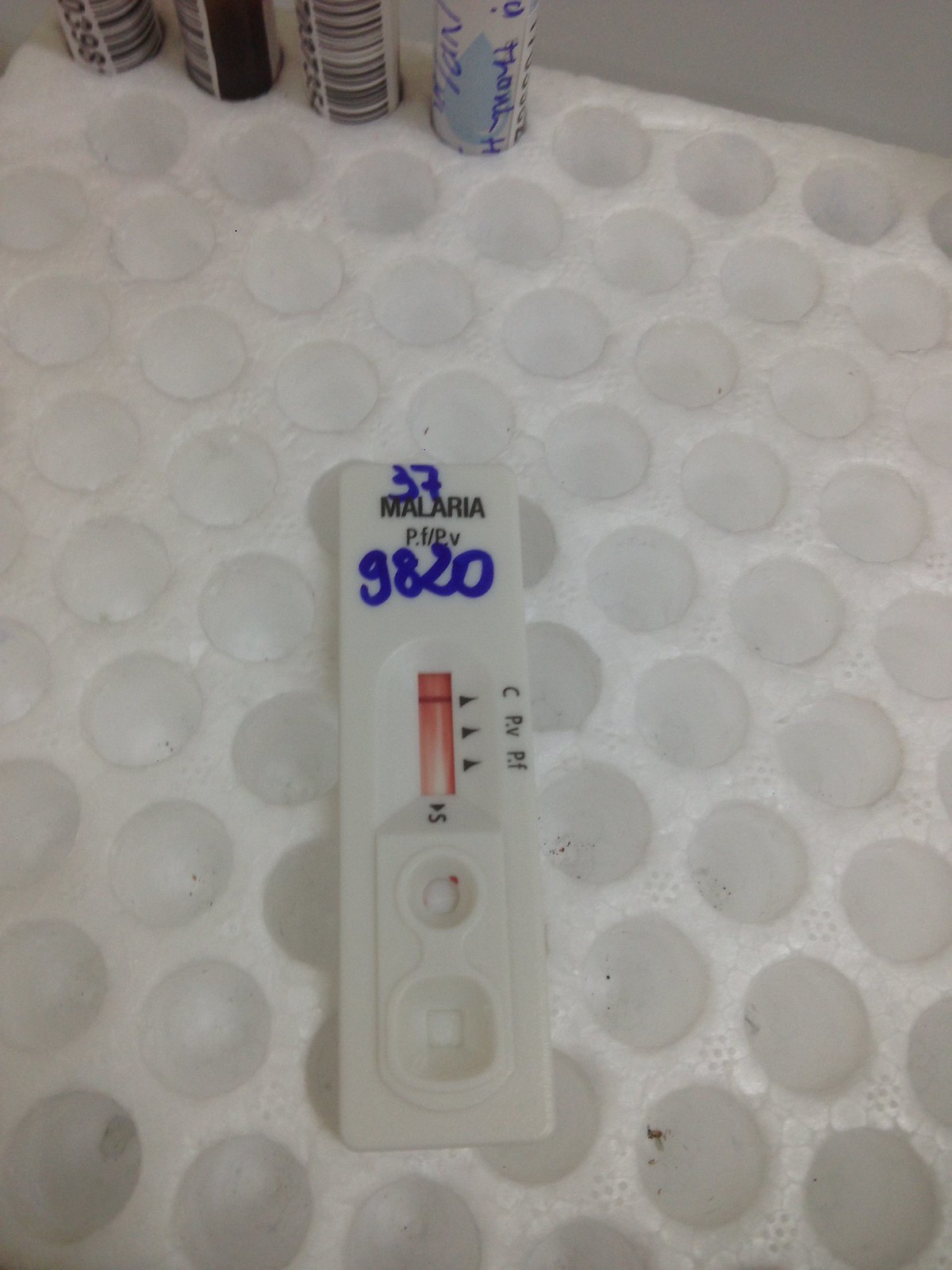The close-up photograph depicts a meticulously organized malaria testing setup. Dominating the image is a large piece of styrofoam with numerous uniformly arranged holes, designed to hold test tubes. At the upper left corner, four test tubes are visible, though partially obscured. The three test tubes on the far left feature black and white UPC labels, while the fourth one, which is slightly rotated, displays a hand-written note. Unlike the other three, this fourth test tube sports a blue and white label. The extensive styrofoam panel, with its 10 to 12 rows of empty slots, extends beyond the frame, suggesting a large-scale testing operation.

Mounted vertically on the styrofoam is a plastic rectangle labeled "malaria" at the top, with "37" handwritten in blue marker above it. Below this, the printed text reads "P. F. / P. V.," and a handwritten notation that appears as "g820" is present nearby. This plastic component includes a recessed, elongated oval window showing pink coloring with three small triangle markers to the right. A black indicator line is positioned at the topmost marker, potentially signifying a result in the malaria test. Additional black text is present on the right side of this oval window, accompanied by further markings at the bottom. Below this section of the plastic rectangle are two white plastic circles, completing the intricate layout.